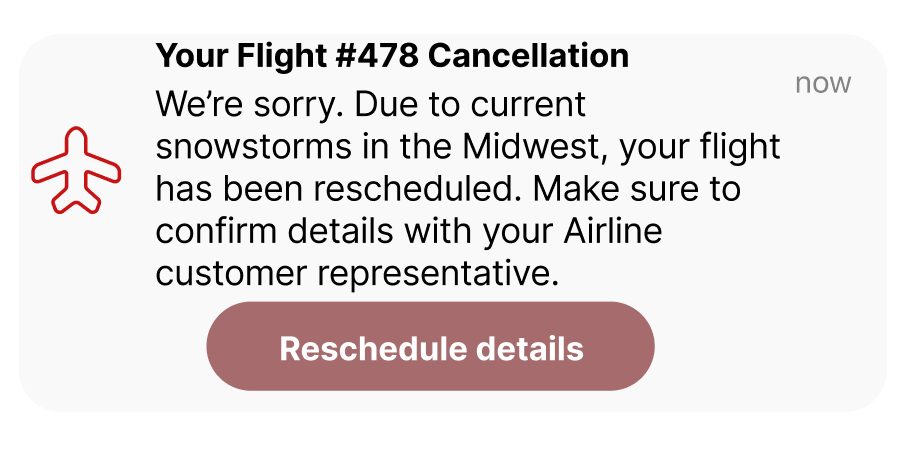The image displays a notification about a flight cancellation against a faint gray background. On the left side, there is a red airplane icon. In the upper right corner, gray letters read "Now," while neon black letters at the top state, "Flight Number 478 Cancellation." Below this, a message in black letters explains, "We're sorry. Due to current snowstorms in the Midwest, your flight has been rescheduled. Please confirm details with your airline customer representative."

Further down, there is a clickable, elongated, oval-shaped button in an off-red color with white letters that say "Reschedule Details." This section allows passengers to find more information about their new flight arrangements. The overall presentation resembles an alert typically received on a phone or a website when a flight is canceled, prompting the user to seek rebooking options. This visual notification mimics the experience of frequent flyers who have encountered similar cancellations in the past.